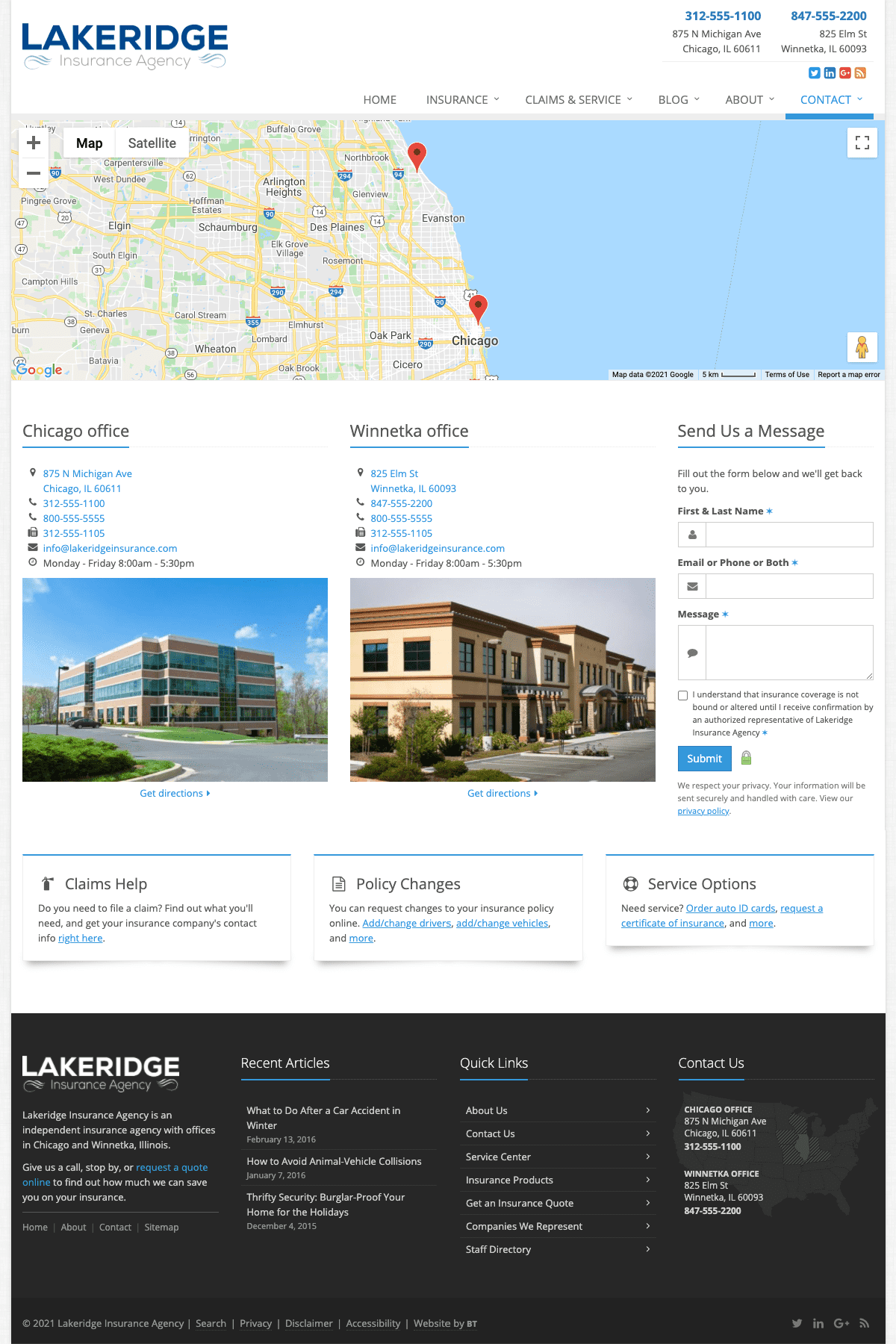The website titled "Lake Ridge" features a detailed map at the top of the page against a blue background, marked with two pinpoints indicating a specific town. Below the map, a section displays the “Chicago Office” heading in underlined black text with a blue line, accompanied by an image of what appears to be an office building. Adjacent to this, another similar office listing is present, though the text is smaller and harder to decipher, but it is also followed by blue font and an associated image of another office building. Towards the side, a "Send Us a Message" section appears, detailing various contact methods in black text. At the bottom of the webpage, a black rectangle prominently displays "Lake Ridge" with four rows of small white text, which are not easily readable.